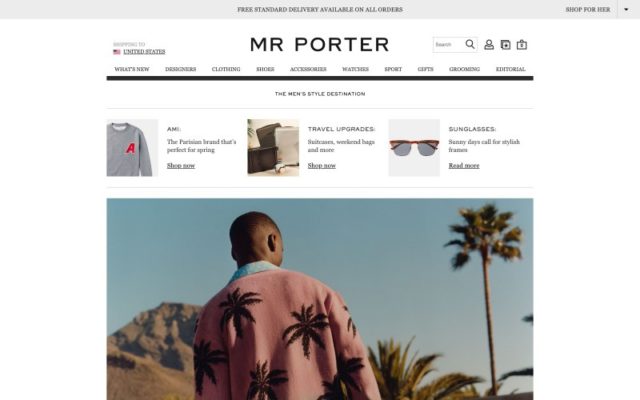The image is a screenshot from a website, likely a fashion retail page. At the top, there is a gray banner with the text "Free standard delivery available on all orders." Immediately below, there's a navigation bar with the "Mr. Porter" logo and country selection marked as "United States." The black submenus include options for "What's New," "Designers," "Clothing," "Shoes," "Accessories," "Watches," "Sports," "Gifts," "Editorial," among others.

The main content area features a series of images. The first shows a gray sweatshirt and is likely a featured product. Another section titled "Travel Upgrades" showcases a set of suitcases. There is also a close-up image of a pair of sunglasses labeled simply as "Sunglasses."

A prominent image features a dark-skinned person outdoors, wearing a pink shirt with a blue collar adorned with brown palm tree motifs. The background shows a clear blue sky, green palm trees, and a brown mountain range. The person is looking off to the side, giving a casual vibe.

To the right of the "Mr. Porter" logo in the navigation bar, there are several icons, including a search box represented by a magnifying glass, a user profile icon, a box icon, and a shopping bag icon. The text in the image is somewhat blurry and hard to read due to zooming, but there are no other notable visual elements.

In summary, the screenshot captures a stylish and minimalistic website interface focused on showcasing men's fashion items along with user-friendly navigation elements.